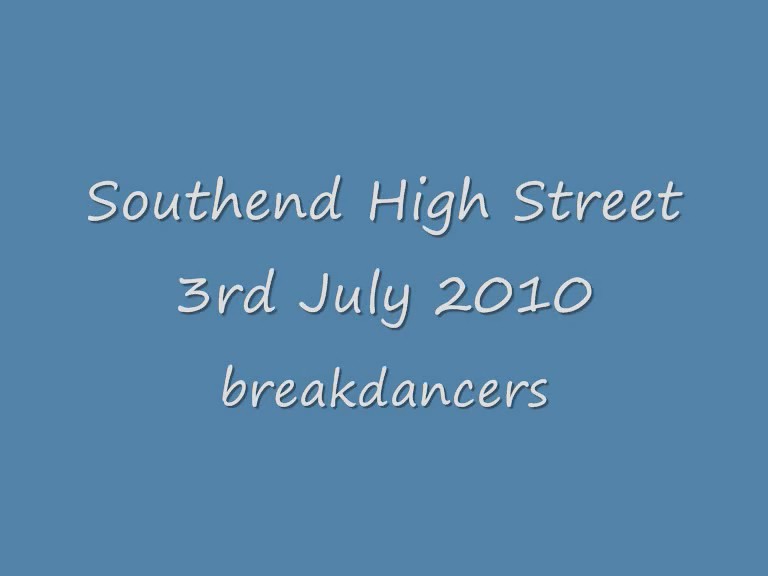The image is a large, light gray-blue poster or screenshot featuring three rows of casual, handwritten-style white text with a dark gray drop shadow effect for added depth. The text is centrally aligned, with generous spacing between each line. The top row reads "South End High Street" in a font reminiscent of comic sans but slightly more cursive. The middle row displays the date in uppercase, "3rd July 2010," and the bottom row, written in all lowercase, simply states "breakdancers." There are no additional images or details on the poster, suggesting that it was likely used as an informational sign or social media post to announce a breakdancing event at South End High Street on that date.